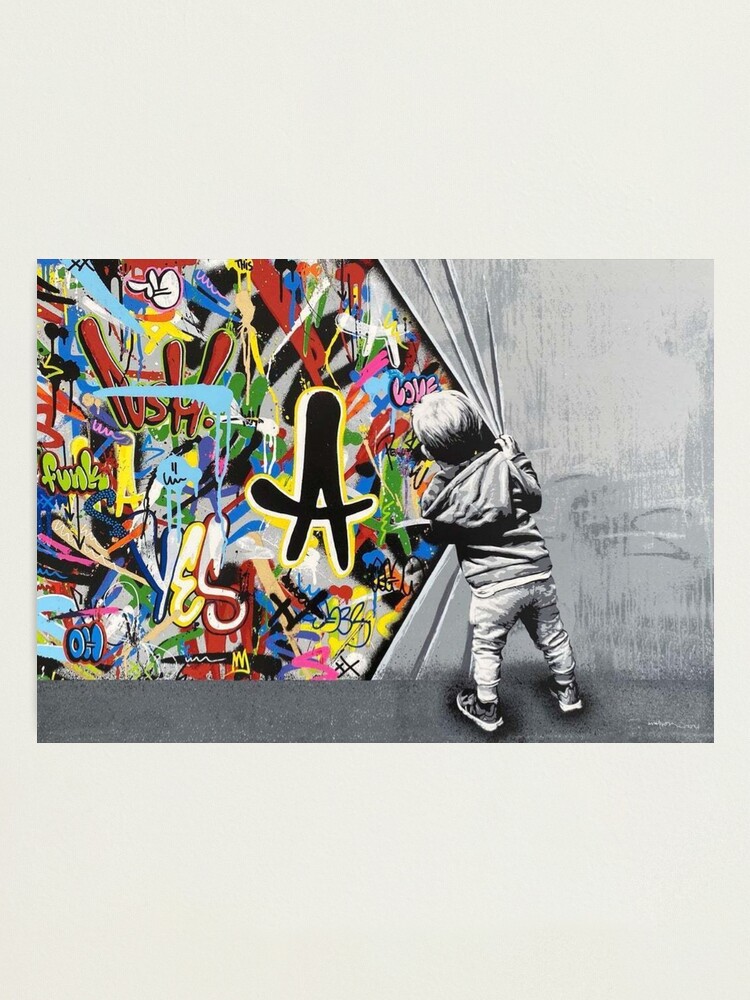The image depicts a young boy, approximately 2 to 6 years old, standing with his back to the viewer. He is dressed in a hoodie, jogging pants, and sneakers, all rendered in black and white. The curtain he is pulling back is also in shades of gray and white, creating a striking contrast with the vibrant scene behind it. This scene bursts with colorful graffiti, featuring an array of words and designs in fluorescent and vivid hues. Notable graffiti elements include the word "funk" in fluorescent green, the letter "A" in black, and the word "yes," with each letter in different bright colors – blue, white, and yellow. The graffiti wall is a chaotic and energetic mix of shapes and colors, including reds, blues, greens, pinks, and yellows, which makes it pop against the monochrome foreground. The overall composition centers the boy, who appears to be standing in awe at the colorful world he has unveiled. The scene is framed with a subtle gray border on the right and left sides, helping to focus the viewer's attention on the central, more dramatic part of the artwork.